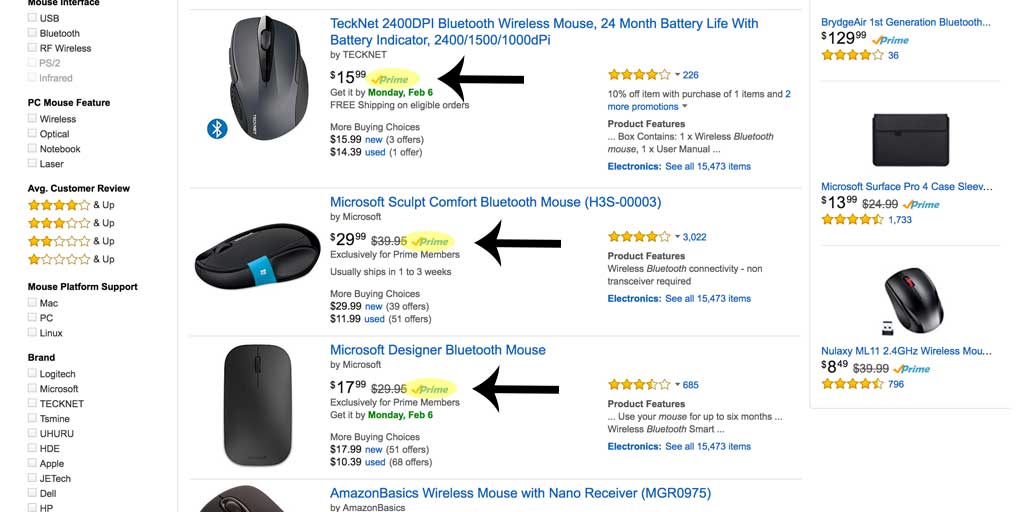This webpage appears to be an online retail platform resembling Amazon, dedicated to the sale of computer mice. The header of the page is not visible, but the central area displays the items for sale, accompanied by a toolbar on the left side. The toolbar offers various selection options based on customer reviews, such as "Four stars and up", "Three stars and up", "Two stars and up", and "One star and up".

The main section of the page features a white background with blue text links next to each item, serving as the pathway to each product's dedicated page. Three different mice are showcased, each highlighted and annotated with additional markings. All three mice are available with Amazon Prime, as emphasized by the yellow-highlighted Prime logos and the accompanying black arrows pointing to the Prime icons.

1. **Top Item:** A TechNet 2400 DPI Bluetooth Wireless Mouse priced at $15.99. 
2. **Second Item:** A Microsoft Sculpt Comfort Bluetooth Mouse listed for $29.99.
3. **Third Item:** A Microsoft Designer Bluetooth Mouse available for $17.99.

The additional annotations and highlights suggest a focus on the Amazon Prime availability of these products, potentially indicating expedited shipping or other Prime benefits.